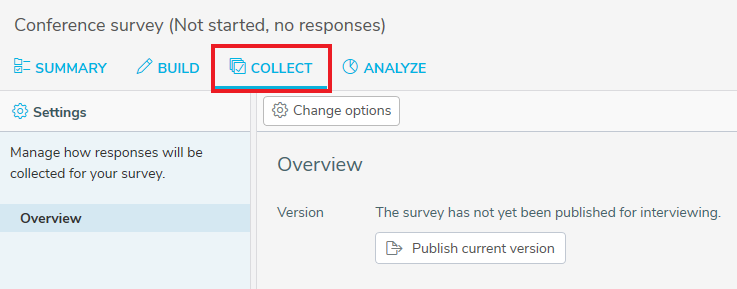Caption: 

"A detailed screenshot of a web page interface, primarily colored in shades of gray, white, black, and blue. At the top is a section titled 'Conference Survey' followed by the status indicator '(Not Started, No Responses)' in black text. The navigation includes several blue-labeled tabs: 'Summary,' 'Files' (with one file checked and two stacked icons), 'Build' (with a pencil icon), 'Collect' (with stacked papers and a check mark, outlined in red), 'Analyze' (with a clock icon), and 'Settings' (with a blue gear icon). A description under 'Settings' reads 'Manage how responses will be collected for your survey.' The 'Overview' option is selected in blue. To the right, another gear icon with the label 'Change Options' is visible in gray. Below, there's an 'Overview' section indicating the survey version status, stating that the survey has not yet been published for interviewing. A button labeled 'Publish Current Version' is displayed, inviting the user to publish the survey."